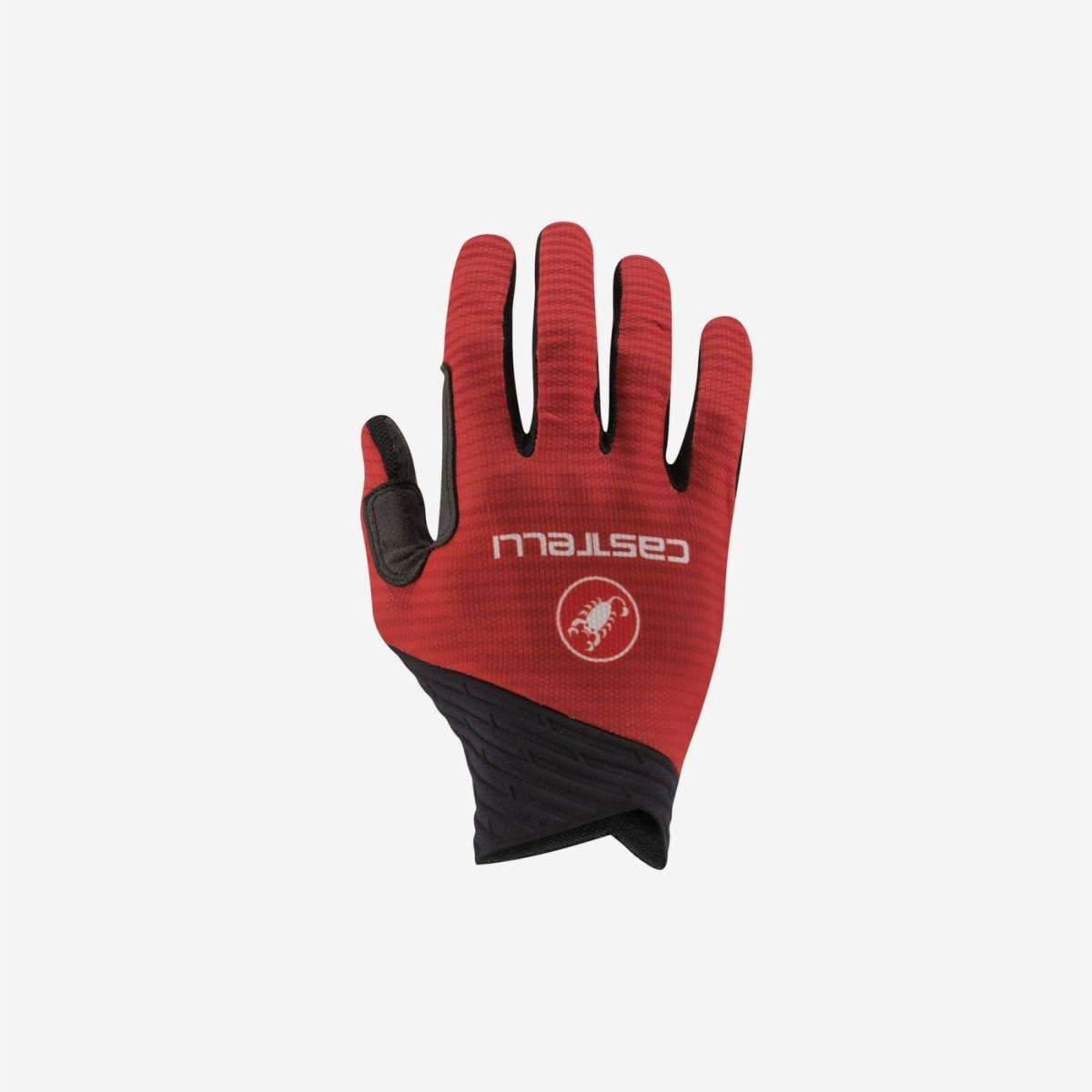This photograph showcases a right-hand cycling glove, set against a plain white background indicative of a commercial catalog or online store. The glove predominantly features a red canvas material on the back of the hand, while the palm, thumb overlay, and wrist sections are constructed from black leather. Positioned with the fingers pointing upwards and the wrist downwards, the glove's branding appears inverted, displaying the name "Castelli" in white text. Below this text, a distinctive brand logo—a white scorpion encircled in red and outlined in white—is visibly printed. The glove seems designed for athletic use, suggesting durability and functionality suitable for extreme sports such as BMX biking.